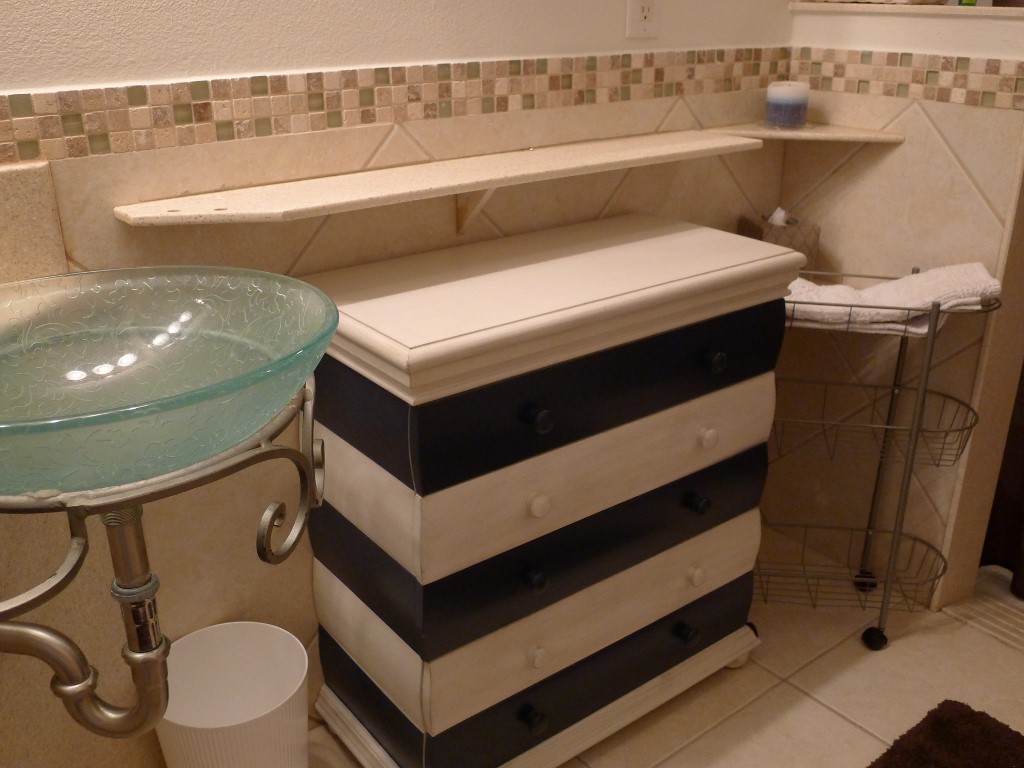The image depicts a meticulously designed bathroom with several distinct features. The floor is adorned with tiles, extending partially up the walls, which are covered in white tiles accented by a border of small square tiles. Above this tiling, the walls are painted and have a heavy texture. Built into the tiled section is a recessed shelf.

Beneath the shelf is a dresser characterized by alternating layers of black and white wood, and it features five drawers, all empty on top. To the left of the dresser stands a small white plastic trashcan, while to the right, a metal towel caddy is visible. Positioned in the corner on the left side is a large glass bowl with a drain, serving as the sink, supported by a brass bowl holder. A bath mat lies on the tiled floor, adding a touch of comfort to the space.